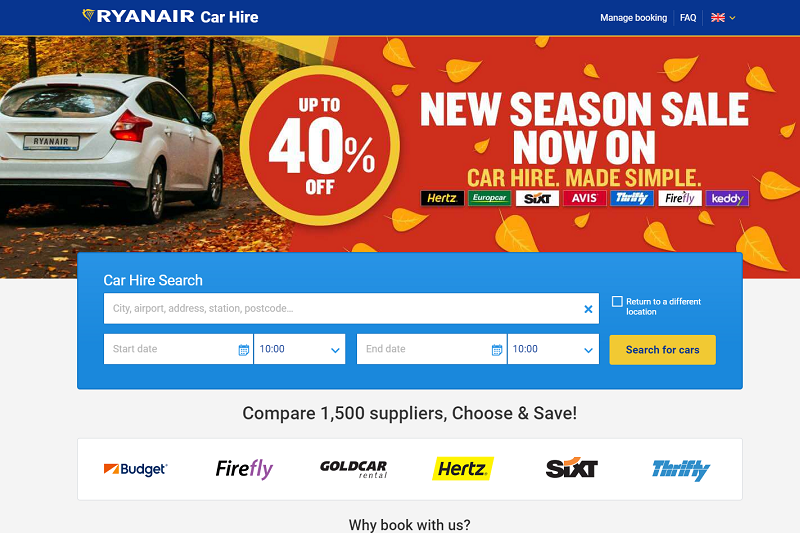This vibrant color advertisement for Ryanair Car Hire, featured on a website, draws the viewer's attention with its autumn-themed visuals and substantial promotional offers. On the left side, the ad prominently displays the Ryanair Car Hire logo, while the right side contains essential navigation options such as Manage Booking, FAQ, and a Union Jack flag indicating language or regional settings.

Central to the ad is a picturesque photograph of a small white car seen from the back, driving along a scenic autumnal woodland road. The license plate displays the Ryanair logo, blending branding with the idyllic image of vibrant fall foliage both in the trees and scattered on the ground.

To the left, a striking red circle surrounded by a yellow border boldly proclaims "Up to 40% off" in white text, highlighting the discount offer. Adjacent to this is a banner announcing the "New Season Sale," with the phrase "Now On Car Hire Made Simple" written in white against a red background, enhanced by falling illustrated leaves, adding to the seasonal theme.

Below these promotional elements, icons of various car rental companies are featured, including Hertz, Europcar, Sixt, Avis, Thrifty, Firefly, and Keddy, providing a variety of options for potential customers.

The lower section of the ad includes a car hire search tool with input fields for the city, airport address, station, and postcode. Users can also select the start and end dates, each complemented by a calendar icon and a 10 o’clock drop-down arrow for time selection. An option to return to a different location or to search for cars is available, promoting convenience and flexibility.

Additional text beneath the search tool emphasizes benefits such as the ability to compare 1500 suppliers and the opportunity to choose and save from various rental services, including Budget, Firefly, Go Car Rental, Hertz, Sixt, and Thrifty. The "Why Book With Us" section likely lists further advantages or assurances, although it isn't detailed in the description.

Overall, this detailed and colorful advertisement powerfully combines visual appeal with comprehensive information to attract and inform potential customers about Ryanair Car Hire services.